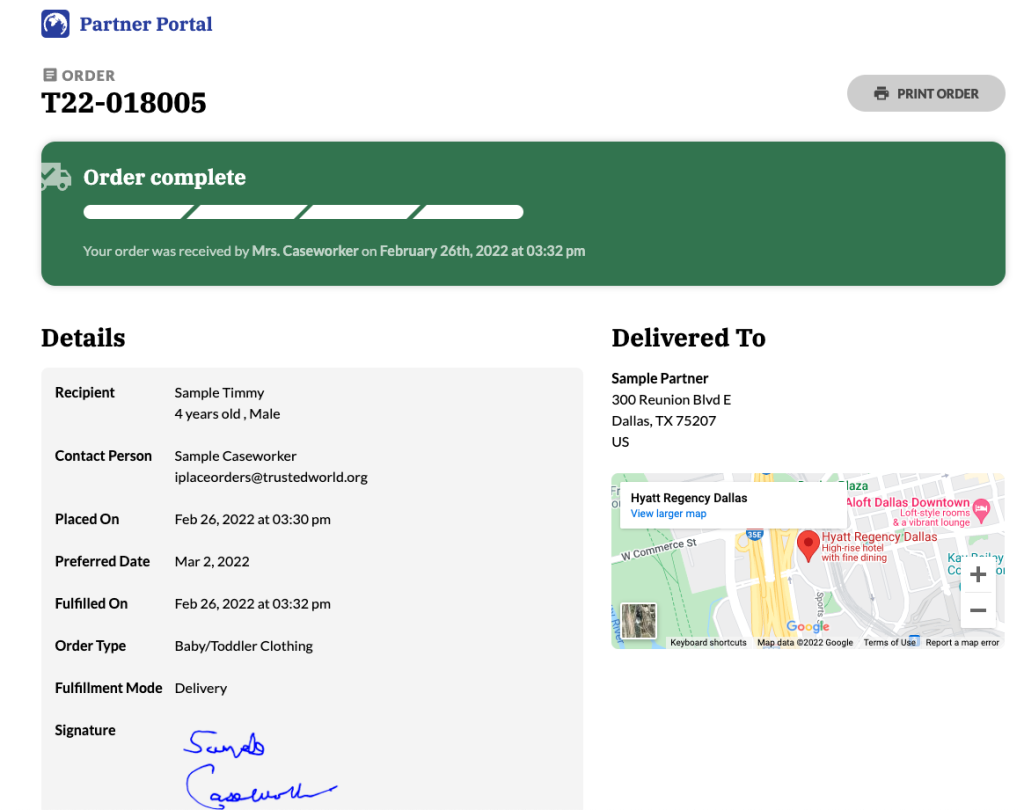A color screenshot in landscape format displays the interface of a platform labeled "Partner Portal," identifiable by its striking blue logo featuring the brand name in capital letters and a stylized globe in white and blue. The focal point of the image is the notification of a completed order, designated as Order T22-018005. The banner "Order Complete" is prominently featured, reiterating the status of the order. According to the details, the order was completed and acknowledged by a Mrs. Caseworker on February 26, 2022, at 3:32 p.m.

The screenshot contains sample data: a four-year-old male recipient named Timmy, and a contact person labeled as 'sample caseworker.' The order was initially placed on February 26, 2022, at 3:30 p.m., and the preferred delivery date was slated for March 2, 2022. Adding a layer of authenticity, the image includes a signature from the individual who finalized the order, along with the delivery address located in Dallas, Texas.

This comprehensive interface overview offered by Partner Portal emphasizes its user-friendly design through placeholders and sample data, intended to familiarize users with the platform's functionalities without exposing actual personal information.